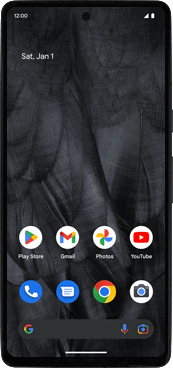The image displays a smartphone screen showcasing various details. The top left corner indicates the time as 12:00, accompanied by a full battery icon and cell reception bars. The date displayed is Saturday, January 1. The phone's background is an intricate, close-up image of overlapping feathers, with the black background accentuating the feather details which might initially give the impression of cracks on the screen.

Several app icons are prominently visible on the screen. The Play Store icon is depicted within a white circle containing a multicolored triangle consisting of green, yellow, red, and blue. The Gmail icon, also within a white circle, features a stylized 'M' in the same colors. The Photos app icon is represented by a colorful pinwheel within a white circle, showcasing red, blue, green, and yellow hues. The YouTube icon appears as a white circle with a red rectangle, inside which lies a white play triangle.

At the bottom of the screen, there are icons for Call, Text, Google, and Photo, and below them is a Google search bar. The search bar has a 'G' on the left side, and to its right are icons for a microphone and what appears to be a camera.